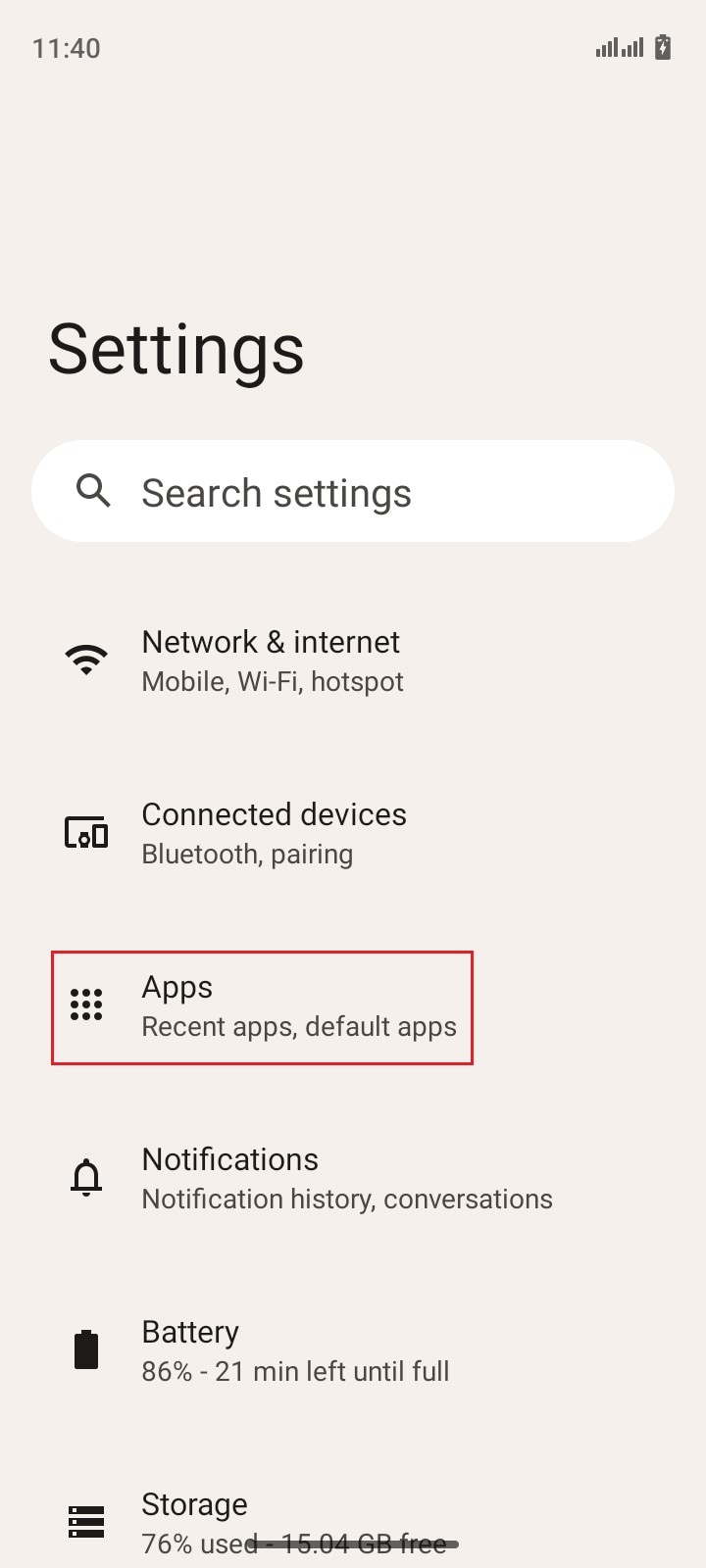Screenshot of an Android device displaying the settings page. At the top of the screen is a search bar with a magnifying glass icon and the placeholder text "Search settings." Below the search bar, various settings categories are listed. 

The first category is "Network & Internet," which includes options such as mobile data, Wi-Fi, and hotspots. Following that is "Connected Devices," featuring Bluetooth pairing options. Next, "Apps" is shown, providing access to recent apps, default apps, and notification settings. 

Additionally, there is a section for "Battery," indicating that the battery is currently at 6% with 21 minutes left until fully charged. The "Storage" section reveals that 76% of storage is used, leaving 15.04 GB free.